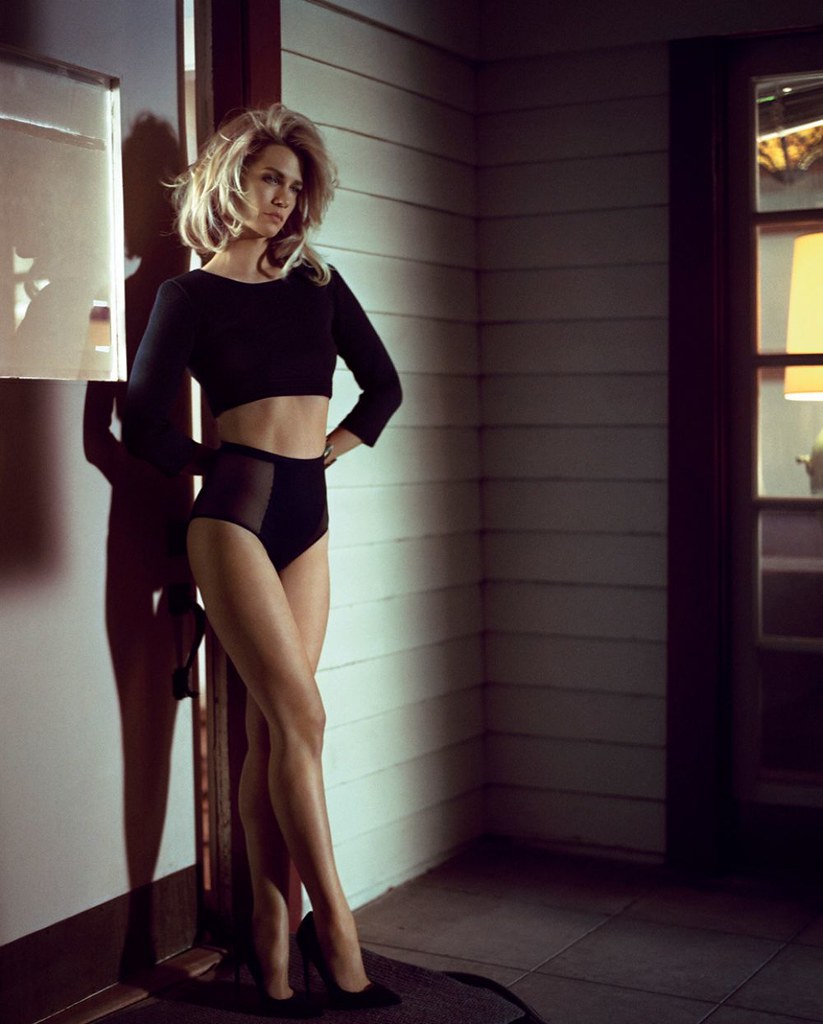In the dimly lit photograph, a young woman in her late 20s stands outside in front of a house. Her medium-length hair is voluminous and poofs out, just above her shoulders. She strikes a slightly angled pose, facing around the three or four o'clock position, with her right leg delicately crossed over her left. Her attire is striking: she wears a long-sleeve black cropped top that reveals her midriff, paired with elegant women's lingerie bottoms made of dark blue, silky fabric with a see-through overlay on her right thigh. The dramatic contrast of the lighting casts her shadow against the house's white siding and door. The scene reveals a bit of the setting's details, including the tile flooring, a carpet towards the bottom left, and additional doorways to either side of the image. The white, wood-paneled exterior of the house and a glimpse of a computer monitor in the upper-left corner add context to the domestic yet intricately set scene, suggesting that the photograph was taken outside the house in the middle of the night.